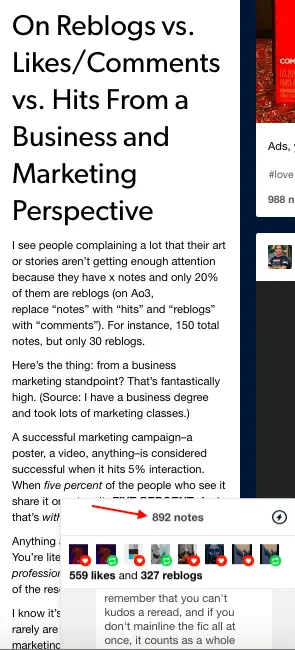This image is a screenshot displayed in portrait mode, capturing only a portion of the screen, notably from the upper right to the lower right. The background is predominantly white, with various elements focused on the differences between reblogs, likes, comments, and hits from a business and marketing perspective.

A notable section of the image, highlighted with a red arrow, draws attention to some statistics and commentary. The text discusses the common complaint among creators that their art or stories aren't receiving enough attention—pointing out that, for instance, if a post has 150 total notes but only 30 reblogs, this kind of interaction is actually quite successful from a marketing standpoint. The creator of the note emphasizes their point by mentioning that they have a business degree and have taken numerous marketing classes, affirming that a 5% interaction rate is generally considered a successful outcome in marketing campaigns.

Part of the text gets cut off, but another highlighted section beneath the red arrow showcases some specific numbers: 892 notes in total, with 599 likes and 327 reblogs. This portion emphasizes another marketing perspective: "Remember that you can't kudos a reread, and if you don't mainline the FIC all at once it counts as a whole." This note points out nuances in how engagement metrics are counted and valued.

Overall, the detailed caption brings forth the idea that from a business marketing viewpoint, even minimal interaction percentages can be considered successful, thus providing a reassurance to creators worried about their engagement rates.